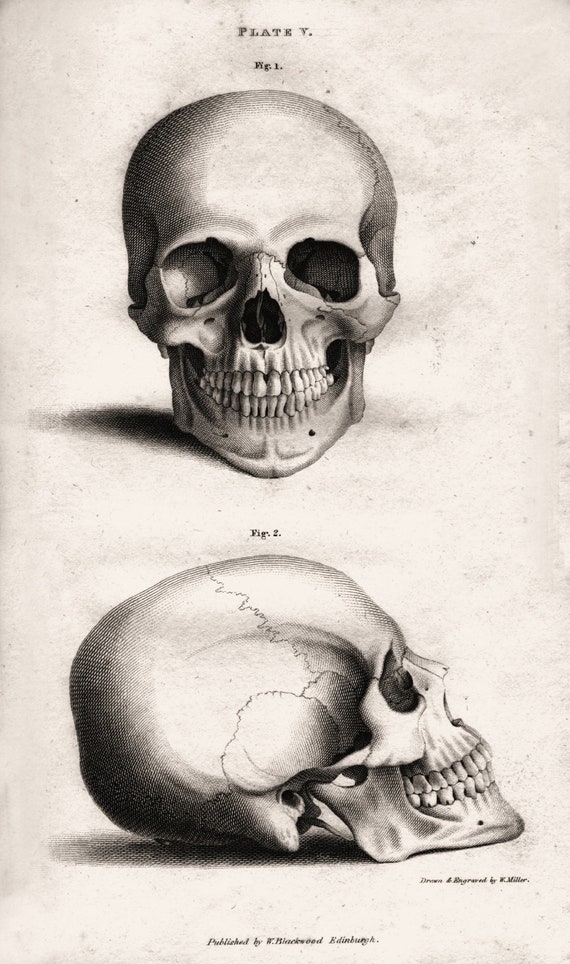This image features a detailed, black and white drawing of a human skull, presented in two distinct views on an off-white background. The illustration is labeled "Plate V" at the top, indicating its place in a series. Both views, one frontal and one side profile, are marked respectively as "Figure 1" and "Figure 2." 

In the frontal view (Figure 1), the skull exhibits pronounced teeth and asymmetrical eye sockets, with the right one being noticeably darker and showing signs of cracking and fissures. The left side of the frontal view is also shaded more heavily than the central region of the skull.

The side profile (Figure 2) illustrates the skull facing right, with noticeable shadowing towards the back. This view highlights a crack running through the skull, beginning from behind the ear and extending towards the rear, implying a significant fracture. Both images suggest a possibly traumatic injury to the skull.

The intricate details of the skull's structure and the labeled figures indicate that this drawing serves a likely educational or medical purpose. The publication information at the bottom reads, "Published by Blackwood, Edinburgh," adding historical context to this anatomical illustration.